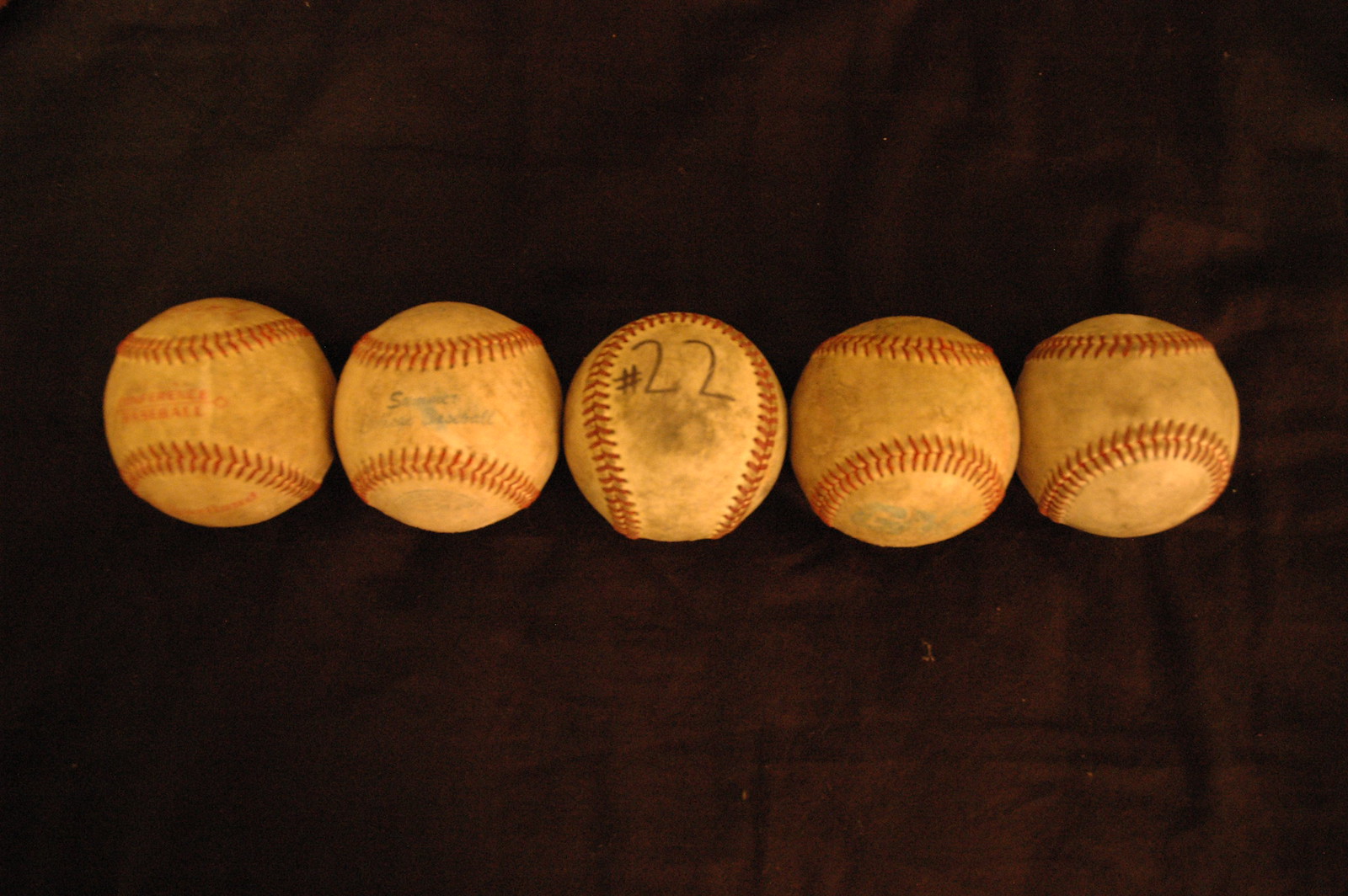This photograph captures a slightly dim view of five well-worn baseballs resting on a brown cloth surface. The baseballs are an off-white, almost beige color, heavily marked with dirt and scuffs, contrasting with their original bright white hue. Each ball features the traditional red stitching, now muted from use, maintaining the familiar patterning. The baseballs are oriented differently, but the ball in the center stands out with its stitching in a horseshoe shape and the number 22 written in faded black marker above it. The baseball on the far left has a red stamp between its stitches, while the one next to it bears a similar faded blue stamp. No visible writing appears on the two baseballs on the right. The overall scene conveys a sense of nostalgia and the rough play these balls have endured.